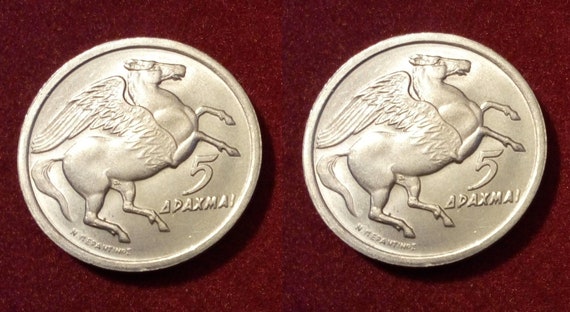This image showcases a top-down photograph of two identical silver coins placed side by side on a deep blood red background, with a small gap between them. Each coin occupies about half of the image. The coins feature an engraving of a Pegasus, a mythical horse with wings, shown in an upright, rearing position with one wing visible due to the side profile. Below the horse's front right leg is the number '5', and directly beneath it is the word 'A-D-A-X-M-A-I'. Additionally, there is some smaller, indistinct lettering underneath the back right leg of the horse.